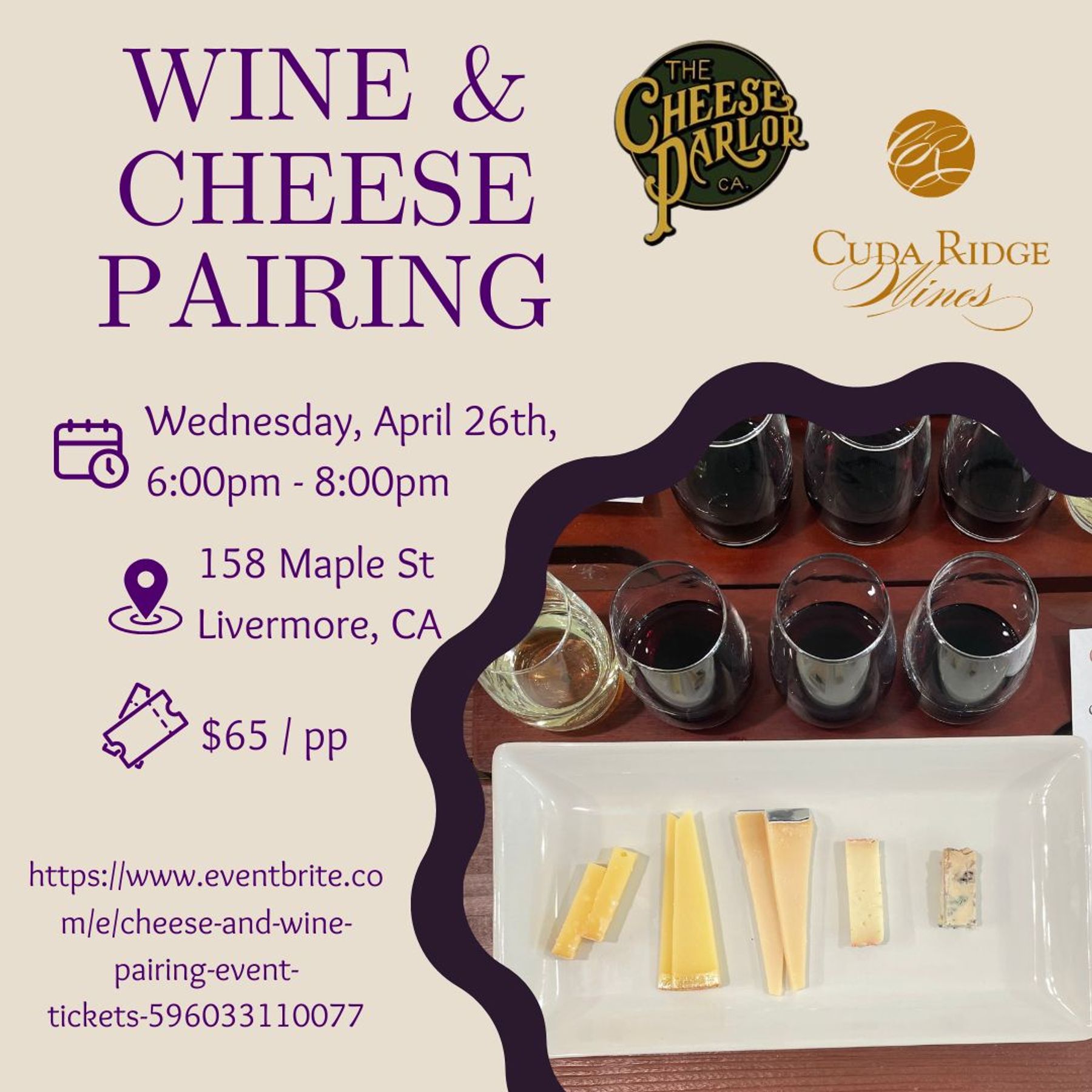This colorful advertisement promotes a Wine and Cheese Pairing event scheduled for Wednesday, April 26th, from 6 p.m. to 8 p.m., at 158 Maple Street, Livermore, California. The event, hosted by Cuda Ridge Wines and The Cheese Parlor, costs $65 per pair. The background of the ad is beige with a dark purple scalloped border in the lower right corner. Central to the design are images of a variety of wines and cheeses: four glasses of wine (three red and one clear) lined up on a wooden surface, and an assortment of cheeses sliced into rectangles and triangles on a rectangular white ceramic plate. The left side of the ad displays the event details in bold blue or purple capital letters, including icons indicating the date, time, location, and ticket price. Contact information is provided at the bottom of the ad. The upper right corner features the logos of Cuda Ridge Wines and The Cheese Parlor.